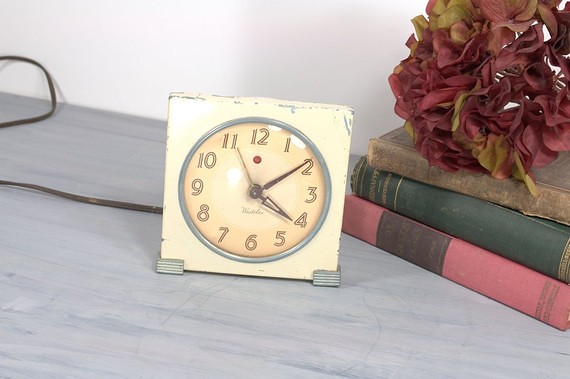This photograph showcases a vintage alarm clock with a distinctly retro design. The clock, primarily square-shaped, features a creamy white casing. Its circular clock face is bordered in a soft blue, giving it a charming old-fashioned flair. The face of the clock has a slightly yellowed tint, indicative of its age. Classic black numerals are elegantly arranged in a traditional 12-hour format, starting from 12 o'clock at the top.

The clock hands comprise a sleek, gold seconds hand and contrasting black hour and minute hands, frozen to display a time of approximately ten minutes past four. This nostalgic timepiece is perched on a stand, which has subtle gray horizontal lines on both the bottom-left and bottom-right corners.

The setting amplifies the clock's vintage appeal, as it rests on a gray desk. Adjacent to it is a small stack of antique books, topped with a delicate arrangement of flowers, adding a touch of timeless beauty to the serene tableau.